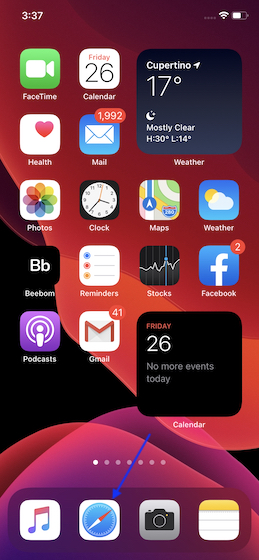This is a screenshot taken from a smartphone, showcasing a colorful background featuring gradient shades of red and purple, blended with an area in black. At the bottom of the screen is a dock containing four icons: a music icon, the Safari icon (depicted as a blue circle with a red and white compass arrow), a camera icon, and the Notes icon (illustrated as a lined piece of paper with a yellow top band). A thin blue arrow points directly at the Safari icon.

Above the dock, the main screen is organized into five rows of smaller app icons and two larger widgets. In the upper right corner, there is a weather widget displaying current weather information. The lower right corner features a calendar widget. The app icons present on the screen include: FaceTime, Calendar, Health, Mail, Photos, Clock, Maps, Weather, BeeBum, Reminders, Stocks, Facebook, Podcasts, and Gmail.